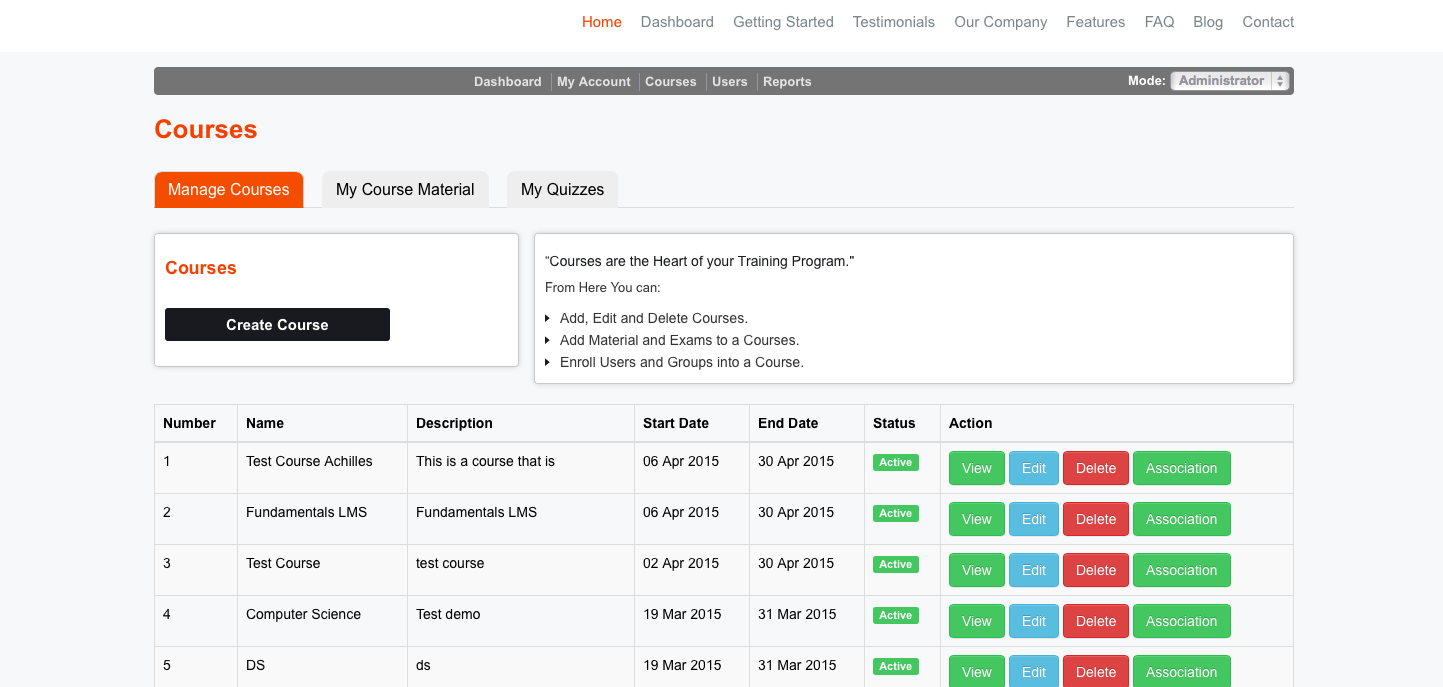Screen capture of an online education platform displaying a class schedule interface. At the top, the navigation bar includes options such as "Manage Courses," "My Course Material," and "My Quizzes." The main content area lists various available courses along with their respective start and end dates. Some of the identifiable course titles include "Computer Science" and "Test Course," while others are too small to read clearly. The platform appears to be designed for signing up for online video lectures or distance learning opportunities.